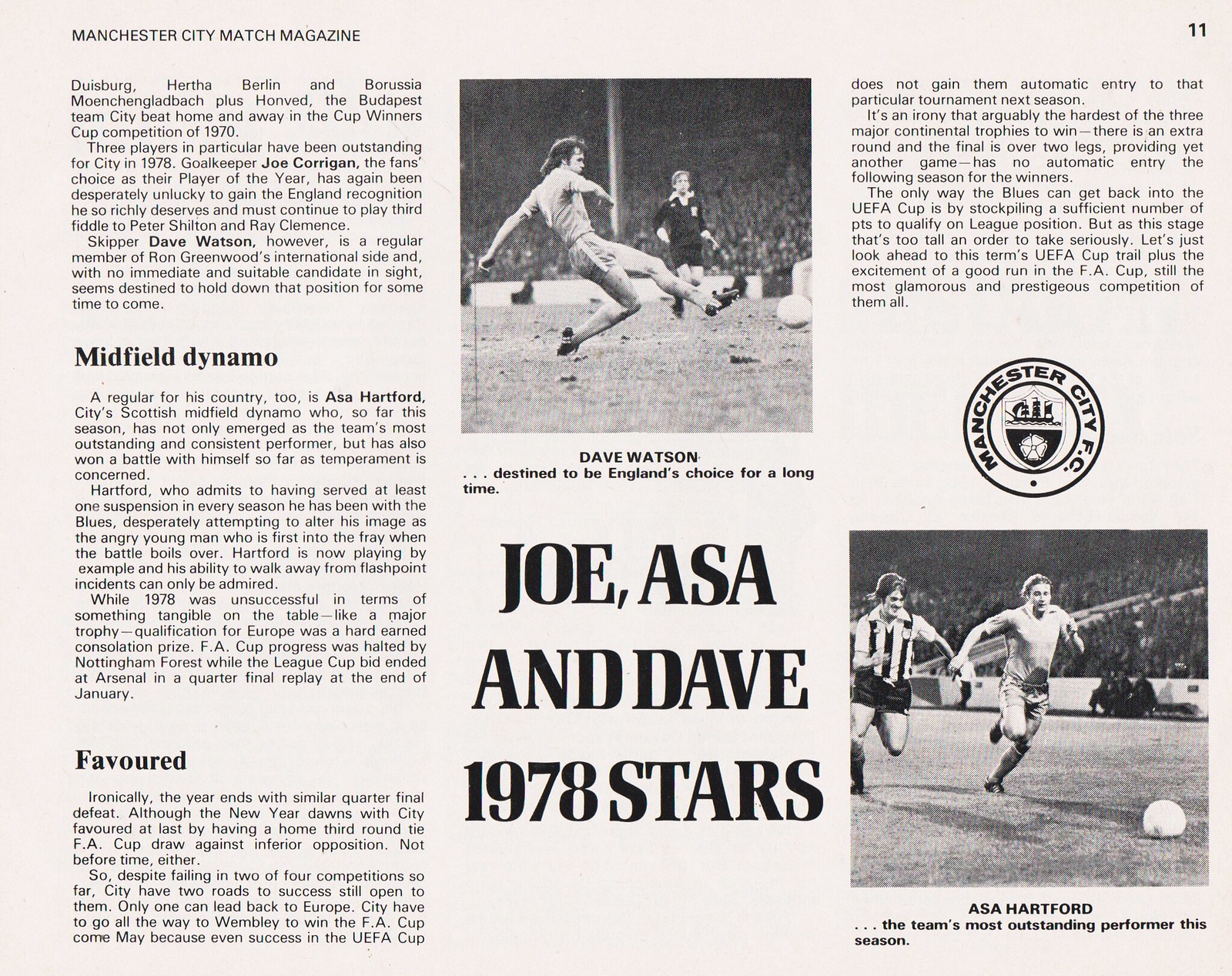The image depicts a scanned page from the Manchester City Match Magazine, specifically page 11, as indicated in the top right corner. The page features a white background tinged with a faint pinkish-red hue and is comprised of three columns of text and photographs.

At the top left of the page, in black font, it reads "Manchester City Match Magazine," establishing the magazine's identity. The left column primarily contains written content, separated by headers such as "Midfield Dynamo" and "Favored," discussing various players and their styles of play. The print is dense and relatively small.

The center column is dominated by an action photograph at the top, which spans about one-third of the column. This black-and-white image shows Dave Watson mid-air, kicking a soccer ball with a stadium full of cheering fans in the background. A caption reads, "Dave Watson destined to be England's choice for a long time." Below the photograph, the text mentions, "Joe, Asa, and Dave 1978 Stars," suggesting the page is from a 1978 magazine issue.

The right column contains a section of text at the top, followed by the Manchester City FC emblem in the form of a coat of arms within two concentric circles, prominently displaying "Manchester City FC." Below the emblem, at the bottom of the column, is another black-and-white photograph. This image captures Asa Hartford in a white top, sprinting towards the soccer ball. Another player in a vertically striped top and dark shorts, also chasing the ball, is partially visible on the left side of the photograph. The background again features a densely packed stadium, emphasizing the popularity of the event.

Overall, the page provides a mixture of visual and textual content focused on key players from Manchester City in 1978.